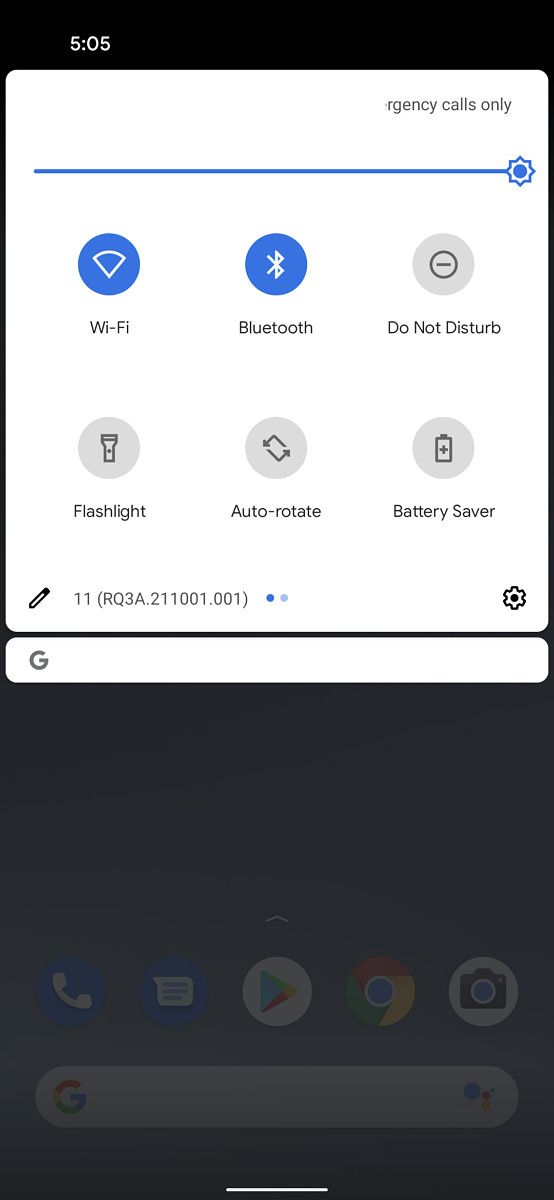The image is a smartphone screenshot captured at 5:05 AM as indicated by the timestamp at the top. In the status bar, the notification "Emergency calls only" is displayed within a white box on the right. The brightness level is indicated by a blue line that is fully extended, showing the brightness is set to maximum. There are several icons in the status bar displaying the current settings: Wi-Fi and Bluetooth are both enabled, while "Do Not Disturb," "Flashlight," "Auto-Rotate," and "Battery Saver" are disabled, indicated by their greyed-out icons.

Additionally, there's a pencil icon and a small number "11" next to a detailed software version listed as "RQ3A.211001.001" in parentheses. On the far right of the status bar sits a settings wheel icon. Below this status bar, the Google logo "G" is visible, suggesting it might be the home screen or Google search bar area.

Behind the white notification box, the smartphone's home screen is partially visible, showing several app icons, including Phone, Notes, Google Play Store, Google Chrome, and Camera. Towards the bottom, a search box with the Google "G" icon to the left can be seen. Although the area is quite dark, it is evident that the screen displays a familiar layout for a smartphone home screen.